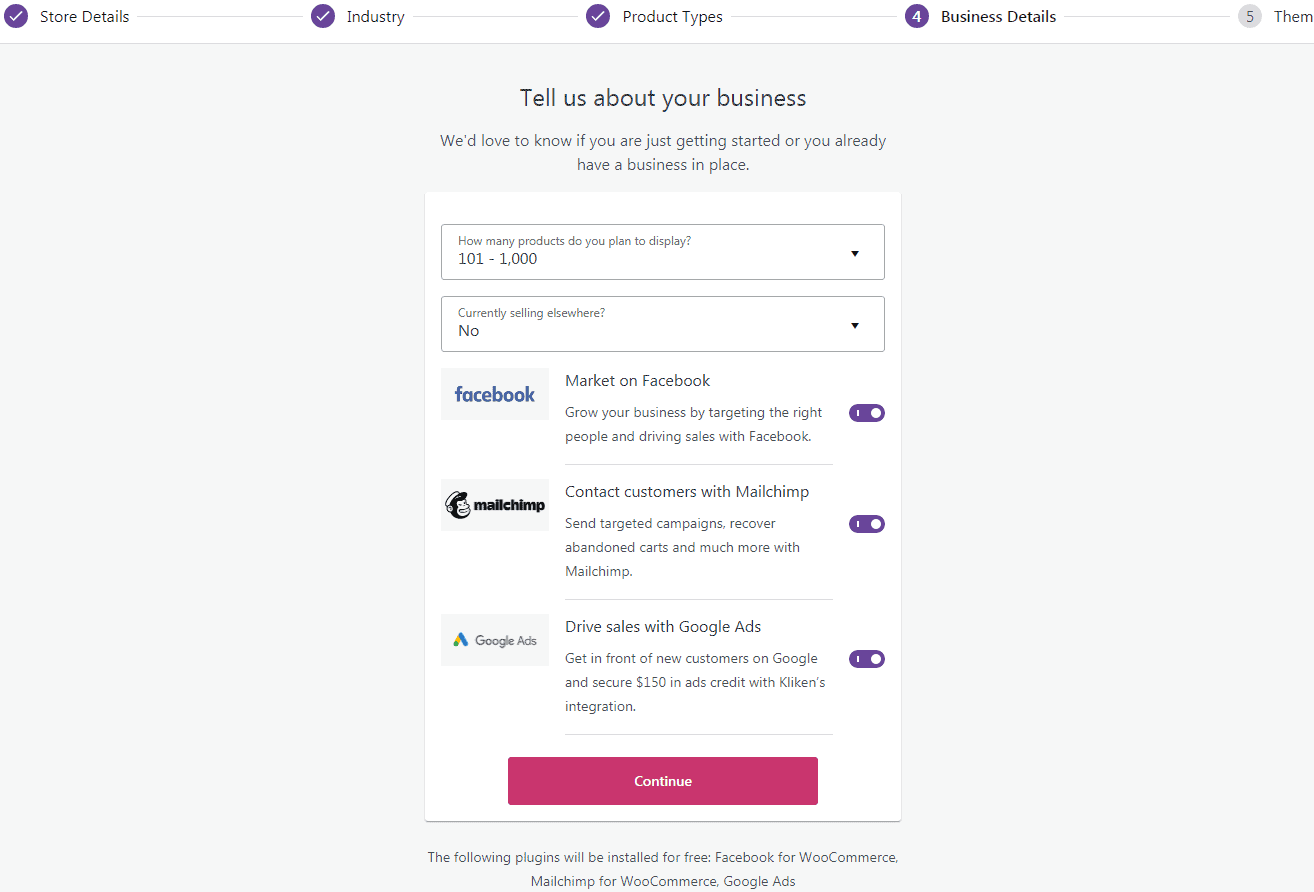This image is a left-to-right horizontal screenshot that you might encounter on a website, computer, or smart device. 

At the top of the image, the background starts with pure white, transitioning into a lighter gray box. The layout features a progression of steps indicated by purple circles with white check marks and numbered icons.

- The first purple circle with a checkmark is labeled "Store Details."
- A connecting line leads to another purple circle with a checkmark labeled "Industry."
- Another line connects to a third purple circle, also with a checkmark, labeled "Product Types."
- The fourth circle contains the number "4" and is labeled "Business Details."
- The fifth and final step is represented by a gray circle with the number "5" and the label "Confirm."

Below this section, the background switches to gray with black text. The header reads, "Tell us about your business," followed by a subheader that says, "We'd love to know if you are just getting started or if you already have a business in place." 

Centered below this text is a vertical white box with a form, starting with the question, "How many products do you plan to display?" The selected option is "101 to 1,000." The form also asks if the user is currently selling elsewhere, to which the selected answer is "No."

Following this, three marketing integration options are presented:

1. **Facebook Marketing** - An icon for Facebook, accompanied by the text, "Market on Facebook. Grow your business by targeting the right people and driving sales with Facebook." This option is toggled on.

2. **MailChimp Integration** - An icon for MailChimp, along with the text, "Contact customers with MailChimp. Send targeted campaigns, recover abandoned carts, and much more with MailChimp." This option is also toggled on with a purple switch.

3. **Google Ads** - An icon for Google Ads, paired with the description, "Drive sales with Google Ads. Get in front of new customers on Google and secure $150 in ad credit with [Kilken's] integration." This option is toggled on as well.

At the bottom of the form, there is a prominent "Continue" button. The footer of the image contains information about various plugins, displayed against the gray background.